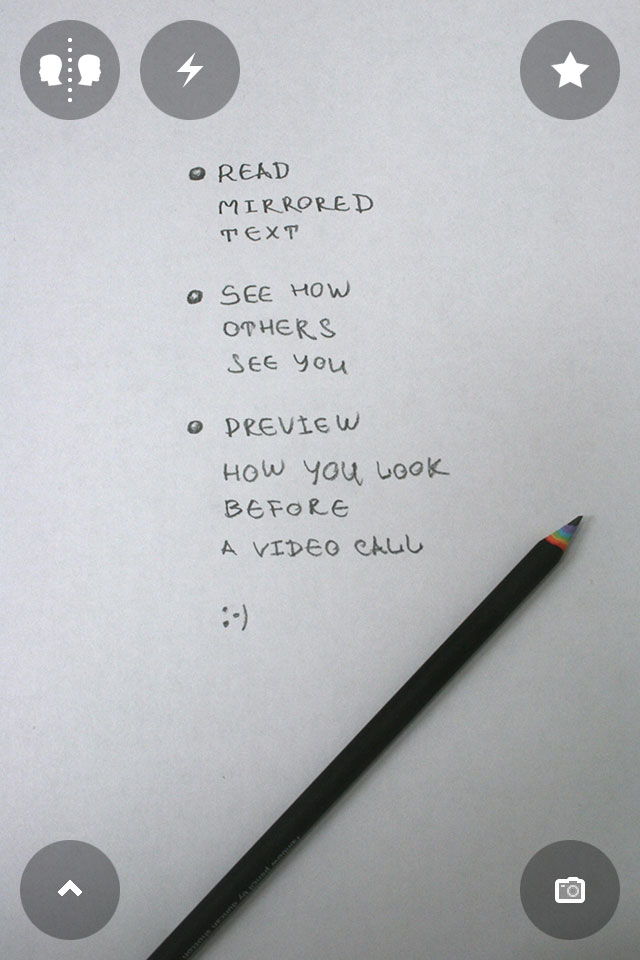The image features a pencil resting on a grayish-white surface. At the top of the image, there are two human head silhouettes facing each other, separated by a dotted line. Below them is a circle with a lightning bolt inside it. In the upper-right corner, there is a white star within a gray circle. Moving to the bottom-right corner, there's a camera icon enclosed in a gray bubble. Directly to the left of this, an upward-pointing arrow is visible in another gray circle. 

In the center of the image, several handwritten bullet points can be seen:

1. Read mirrored text.
2. See how others see you.
3. Preview how you look before a video call.

Additionally, there is a drawn smiley face under these points. Lastly, a colored pencil, primarily black with a blue tip, lies diagonally across the image.